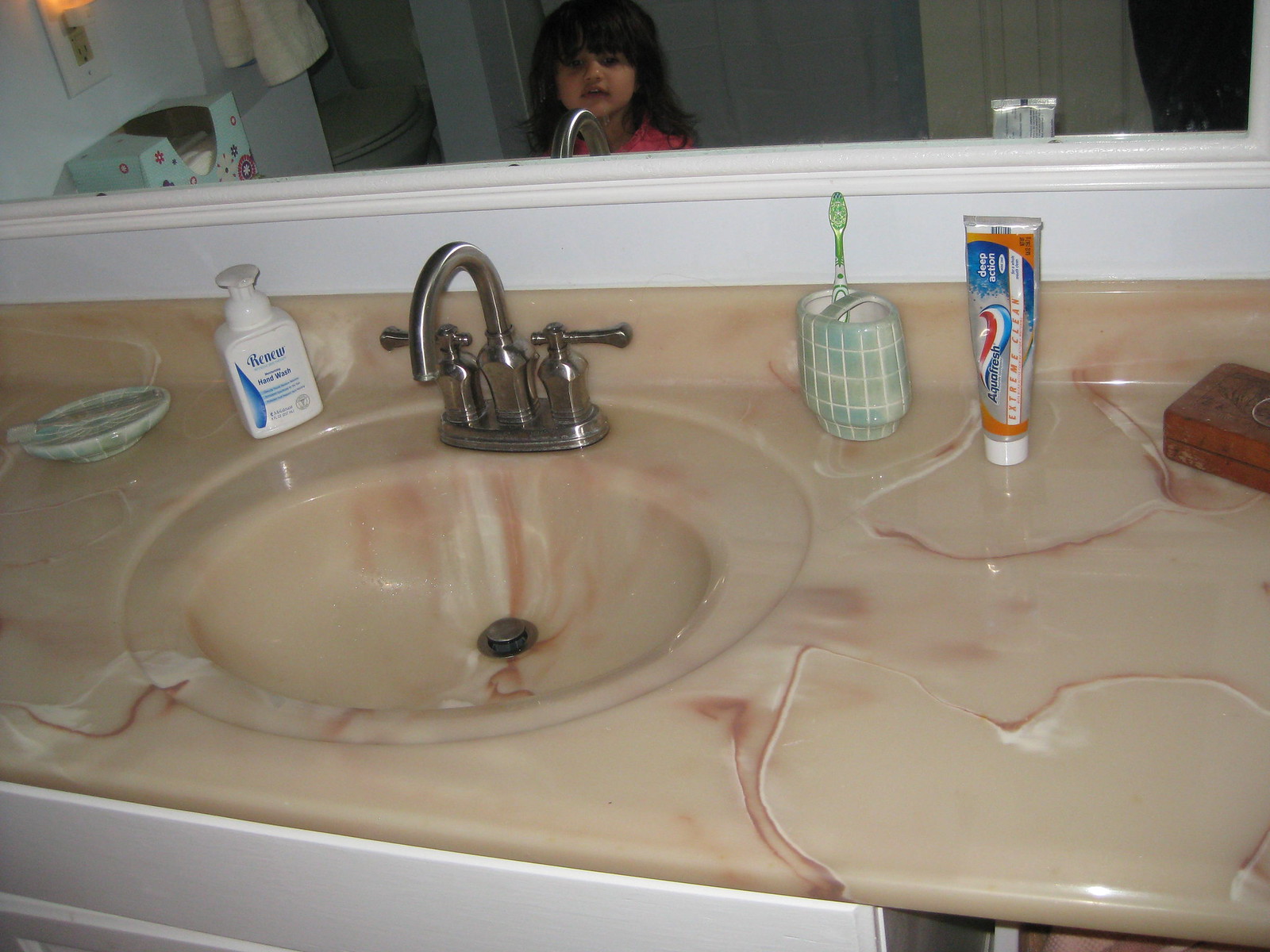In this charming image, a young girl with shoulder-length brown hair is standing in her parents' bathroom, gazing at her reflection in the mirror. She is wearing a pink shirt, and her reflection shows her positioned right in front of the water faucet. Behind her, there is a toilet and a shower curtain. The mirror is mounted above a white panel wall, reflecting the sink and countertop area below.

The countertop itself is a beige color with streaks running through it, featuring a special design. On the counter, there is a green toothbrush holder with a green toothbrush, a tube of Aquafresh toothpaste, a soap holder, and a bottle of hand wash labeled "Renew." Additionally, there is another small green tray. The white cabinets underneath the countertop add to the clean and organized appearance of the bathroom.